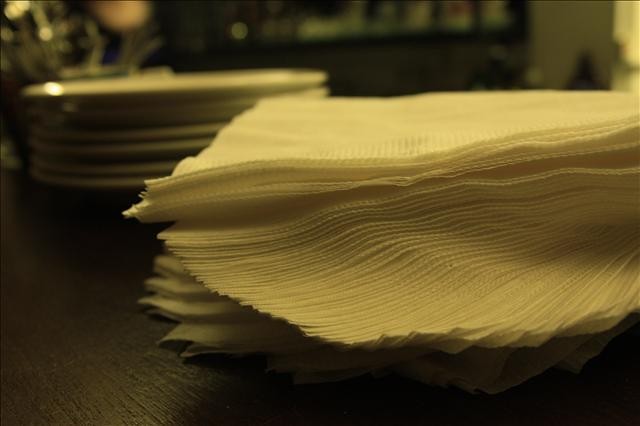The image captures a detailed scene, likely set in a restaurant, although it could potentially be a home dining area. The foreground prominently features a large, slightly tipped-over stack of white paper napkins with a textured top and embossed edges, adding a touch of elegance. These napkins are arranged on a dark brown table, casting noticeable shadows due to its depth of color. Just behind the napkins, a neatly organized stack of white china plates is visible. The table itself is characterized by its dark, almost non-rustic wood grain. In the background, you can discern fixtures typically found at a bar, possibly for pouring beer or soda, adding to the ambiance of a commercial dining space. A brown cabinet can also be seen, holding the plates and other items, partially illuminated to give further context to the setting.